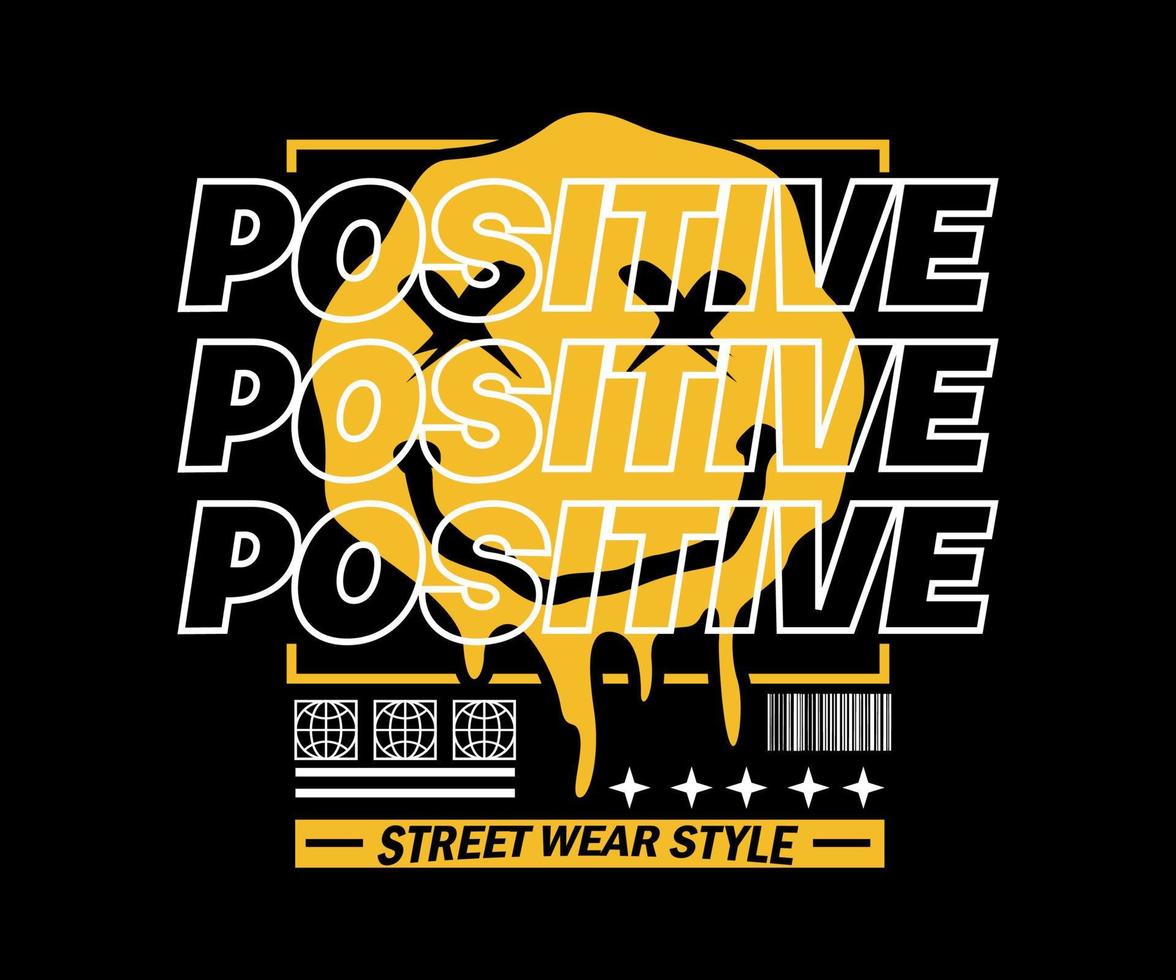This image serves as an advertisement for a streetwear brand. It features a striking design on a solid black background. Dominating the center is a mustard yellow, dripping smiley face with X's for eyes and a wobbly smile, giving a melting effect. Superimposed over this smiley face is the word "POSITIVE" written three times in capital letters, with a see-through effect showing the smiley face beneath. Below the smiley face are three white globe icons, underlined by two horizontal yellow lines. Above this arrangement are five four-point white stars, accompanied by a barcode-like insignia. Completing the design is a bold yellow banner at the bottom, displaying the text "STREET WEAR STYLE" in black capital letters. The overall aesthetic combines vibrant colors and dynamic elements, creating a visually engaging representation of the brand's streetwear ethos.